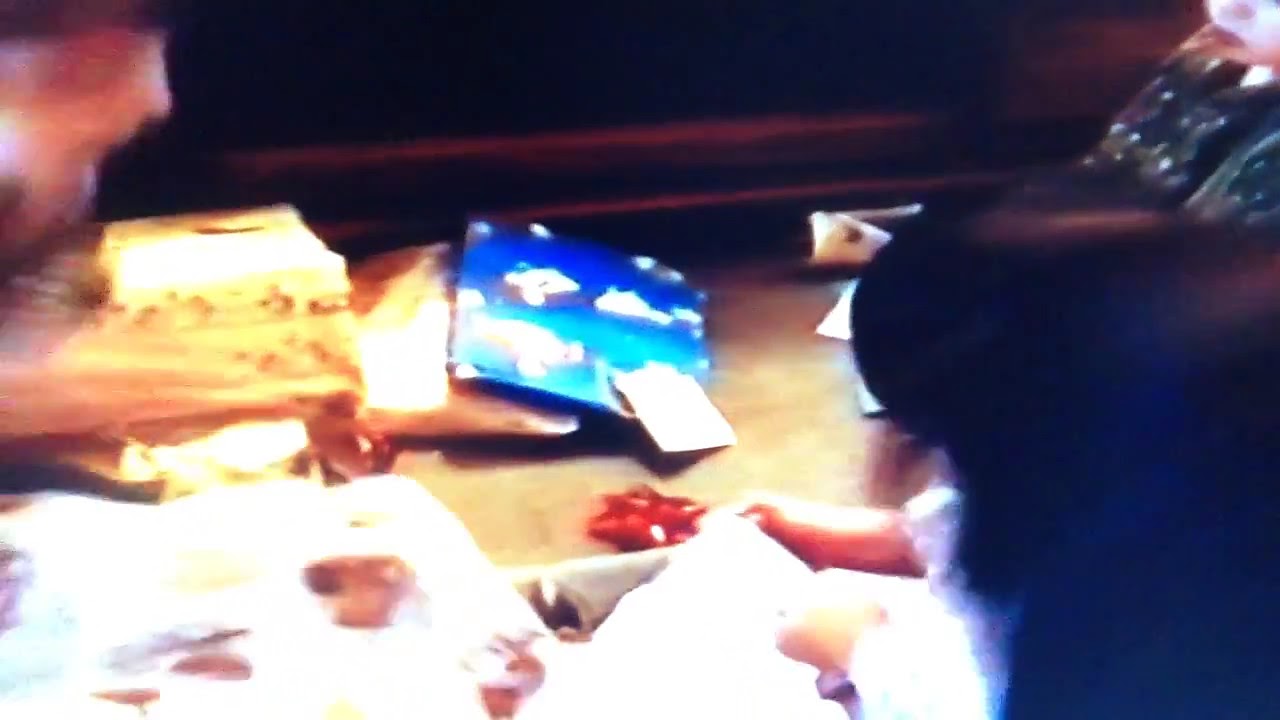In this blurry photograph, a living room scene features what appears to be a little girl with dark hair opening presents on or near a cluttered table. She is partially visible, wearing a white shirt, with her arms engaged with wrapping paper. Surrounding her are an assortment of gifts and gift bags, including a notable blue gift bag with indistinct figures and a shiny red ribbon or bow suggesting a birthday celebration. Various colors of wrapping paper—blue, yellow, red, white, and a couple of rolls of reddish gold—are scattered across the surface, adding to the festive atmosphere. On the right side of the image, a person's face, possibly belonging to someone wearing a green shirt, oversees the activity. Behind the gifts and clutter, there appear to be pieces of firewood arranged on a stand, contributing to the cozy ambiance of a living room, with a wall and some brown trim in the background.